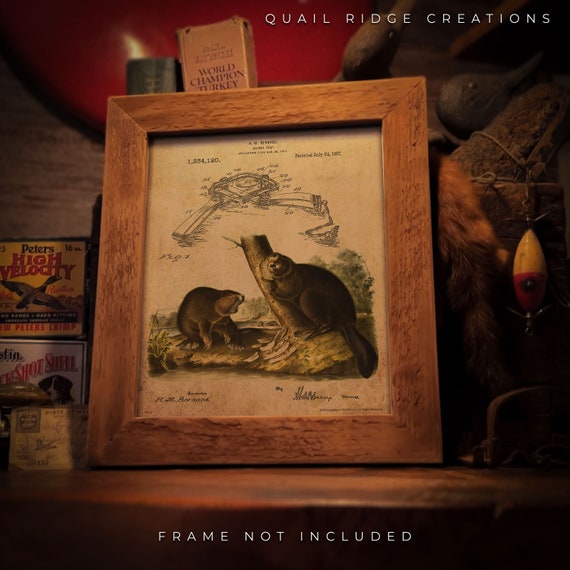The image showcases a detailed drawing of two beavers reminiscent of an old Victorian natural sciences sketch, depicting them standing on a log and chewing the bark off a tree while constructing a dam. The illustration includes schematic elements, possibly a patent drawing, adding to the scientific aesthetic. The sketch, contained within a square wooden frame, bears visible text: "Quail Ridge Creations" at the top right and "Frame Not Included" at the bottom center. The framed artwork is displayed on a wooden table or shelf, which seems to be located in a rustic setting, possibly an old cabin or country store. Surrounding the sketch are various items: to the left, two boxes labeled "Peter's High Velocity," likely containing ammunition, and to the right, a fishing line or bobber. Behind the setup, a bright red wall is visible, as well as an old book titled "World Champion Turkey," adding to the vintage atmosphere of the scene.